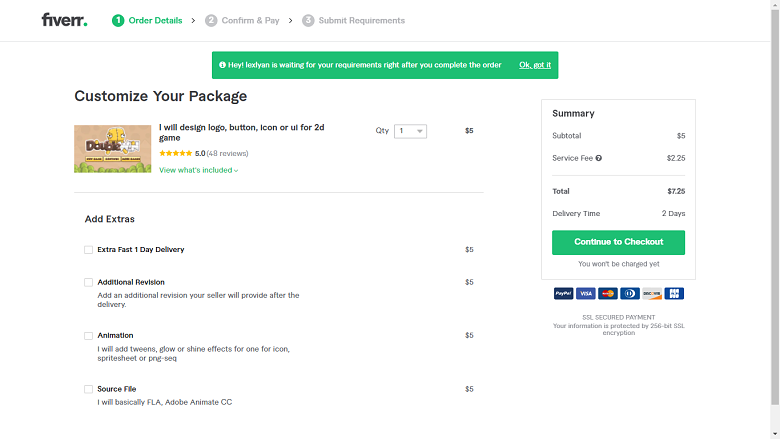The image depicts the checkout section of Fiverr, a popular freelance services platform. At the top right, the word "Fiverr" is prominently displayed. Below this, there are three distinct tabs titled "Order Details," "Confirm & Pay," and "Requirements," with arrows connecting them to indicate the sequence of steps to complete the order.

In the main section, there's an option to customize the package with a specific service description: "I will design a logo, button, icon, or UI for a 2D game." The service is priced at $5, and it has received 48 reviews. 

To the right, a summary box tallies the costs, including a subtotal, an additional service fee, resulting in a total of $7.25. Options for extra services are listed below, such as expedited one-day delivery, additional revisions, or animation services.